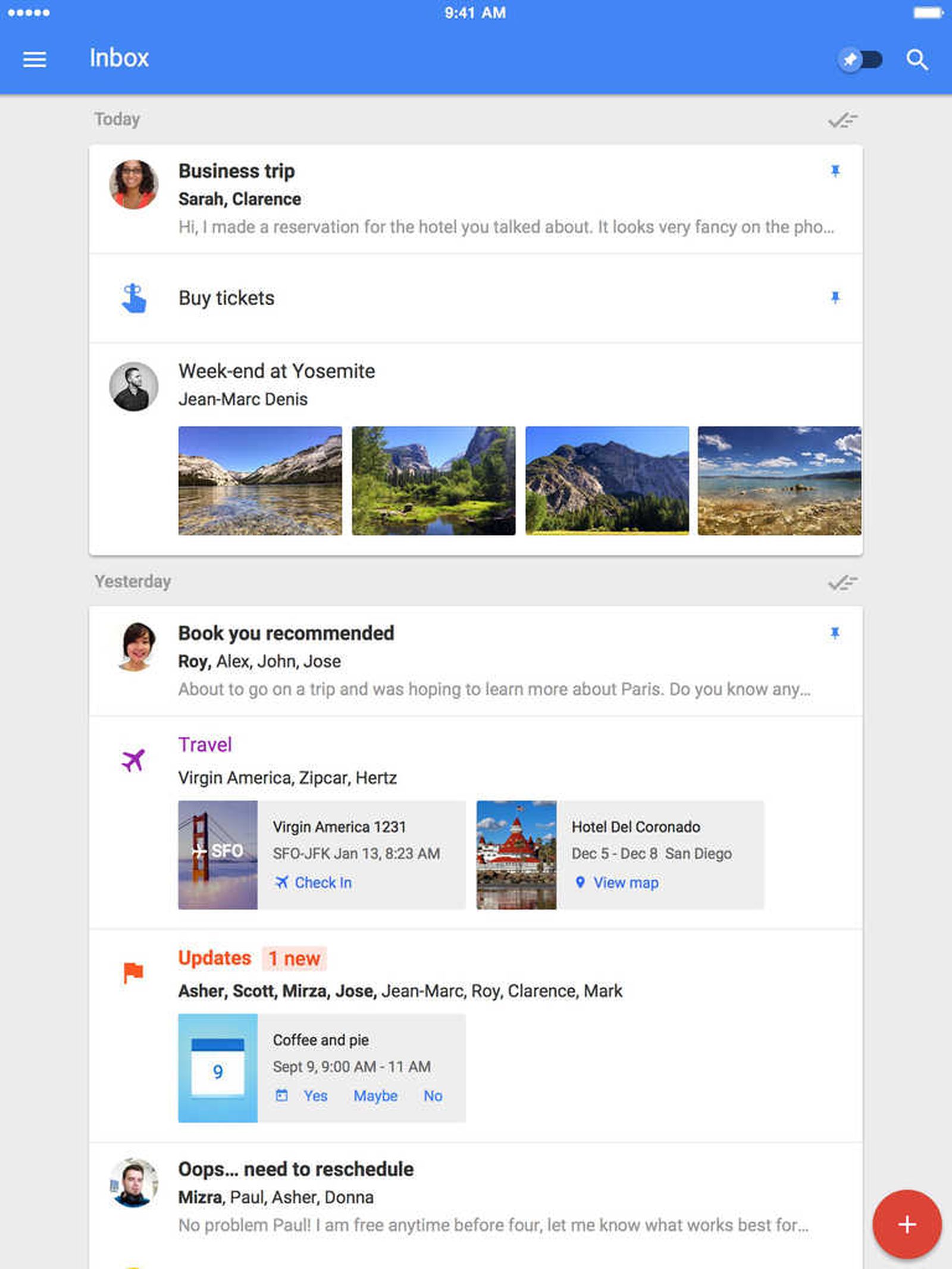A computer screen displaying an email inbox interface. At the top, there's a navigation bar featuring a pin icon and a magnifying glass on the top right. The inbox is segmented by dates, with the first section titled "Today." Below this header, there's an email from "Sarah Clarence" regarding a business trip with a brief preview stating she made a hotel reservation. This email includes a small picture of Sarah Clarence. Following that, there's another email with an action button labeled "Buy Tickets," indicated by a blue hand icon and a pin next to it.

The next section is titled "Yesterday" and features an email about a book recommendation from "Roy Alex." There's a preview mentioning Roy needing more information about Paris, along with a thumbnail image of a woman. This is followed by a list under the heading "Travel" that includes logos for Virgin America, Zipcar, and Hertz, along with a small image of the Golden Gate Bridge. Details for a Virgin America flight (Flight 1231 from SFO to JFK on January 13th, 8:23 AM) and a hotel reservation at Hotel Del Coronado in San Diego from December 5th to December 8th are also shown.

The section titled "Updates" lists events and notable mentions, including an event titled "Coffee and Pie" scheduled for September 9th from 9 AM to 11 AM, with participants including Asher, Scott, Merza, Jose, Jean Marc, Roy, and Clarence Marc. A follow-up message mentions needing to reschedule the event. Additionally, a message reads, "No problem," from Paul, indicating availability before 4 PM.